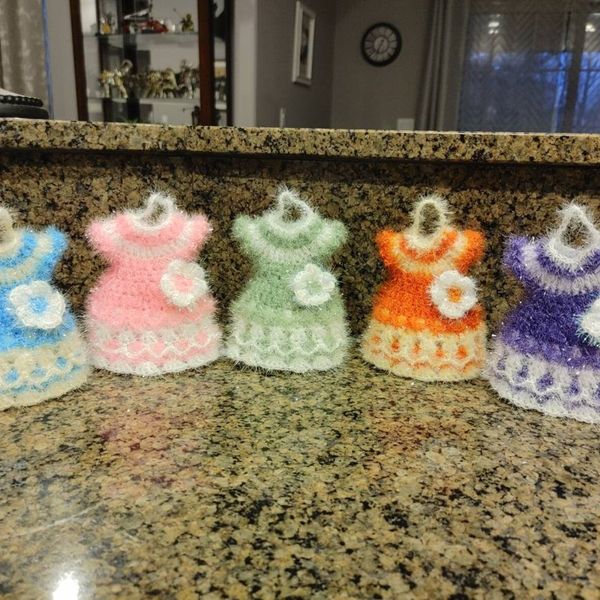The image is a color photograph in a square format showcasing five intricately crafted doll dresses. These dresses, made using cross-stitch techniques, are displayed side by side on a granite countertop in a kitchen, with a higher ledge behind them. From left to right, the dresses are colored light blue, pink, green, orange, and purple. Each dress features a detailed design with short puffy sleeves, a white motif stitched at the bottom, and a white cross-stitched flower adorning the waistband. They also have white string hangers at the top. The background provides a glimpse into a living room area with open sliding doors, a wall clock, framed art, and a glass cabinet, emphasizing a homely setting. The overall style of the photograph leans towards representational realism, capturing the fine details and vibrant colors of the dresses vividly.